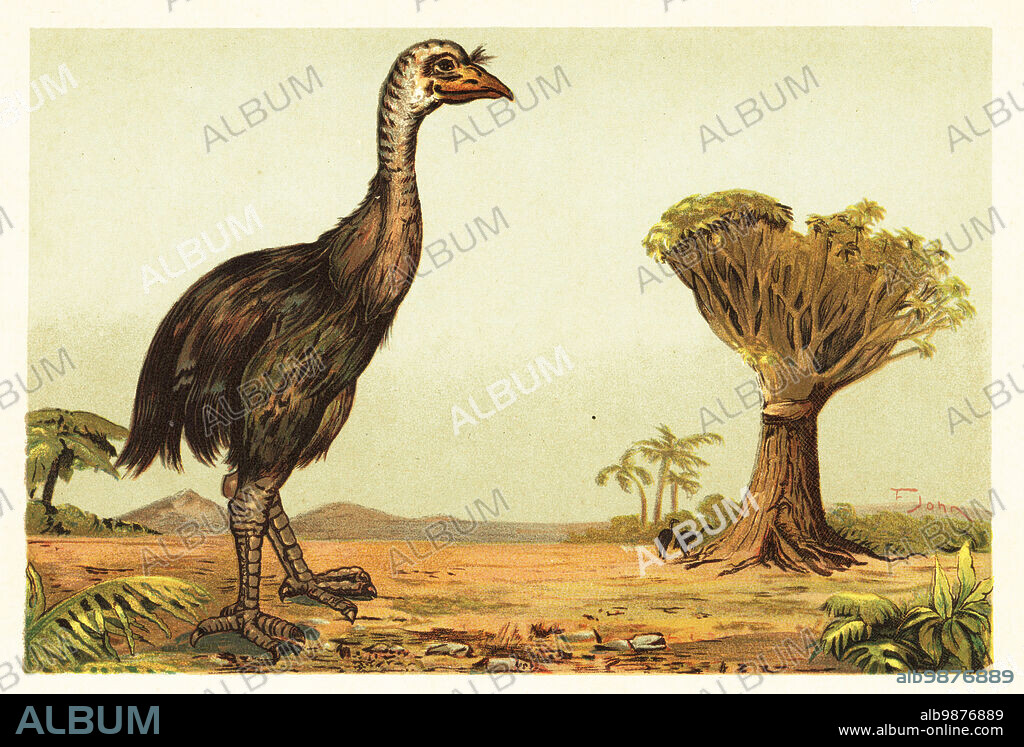This detailed illustration depicts a large ostrich-like bird set in an exotic, likely prehistoric environment. The bird, showing its right side profile, stands prominently in the foreground, featuring a long neck, an orange beak, and dark gray feathers. Its large legs end in webbed feet with prominent claws. Surrounding the bird are various plants, including smaller ground-level flora and taller, sparse trees near the foreground. The background features towering palm trees and other exotic trees, interspersed with mountain silhouettes against a grayish-blue sky. The majority of the landscape appears arid, with a sandy dirt ground. A watermark in gray lettering reading "Album" spans across the image, and the website "www.album-online.com" is listed at the bottom.